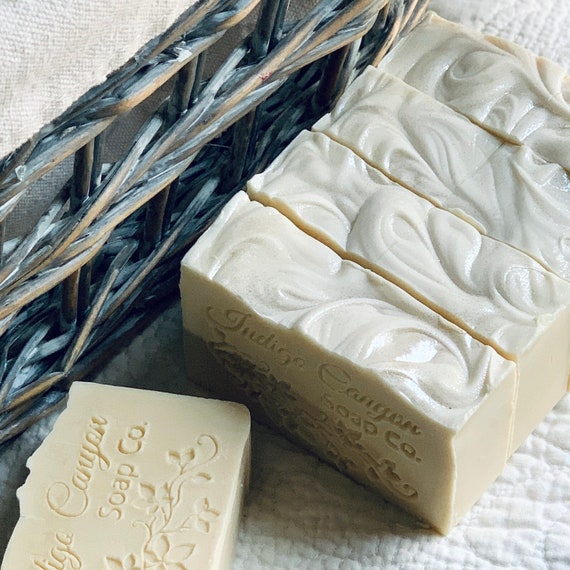This image features five bars of creamy, tan-colored soap, arranged neatly with one bar lying flat while the others are stacked beside it. Each bar displays a distinctive swirled texture on the top, with ridges and uneven details adding to its artisanal appearance. The front of the soap is imprinted with the name "Indigo Cougar Soap Co." and adorned with an intricate design of flowers, leaves, and vines. The soap rests on a white fabric, creating a clean and elegant backdrop that contrasts with the rustic wicker basket placed behind it, which features a mix of black and yellowish colors.